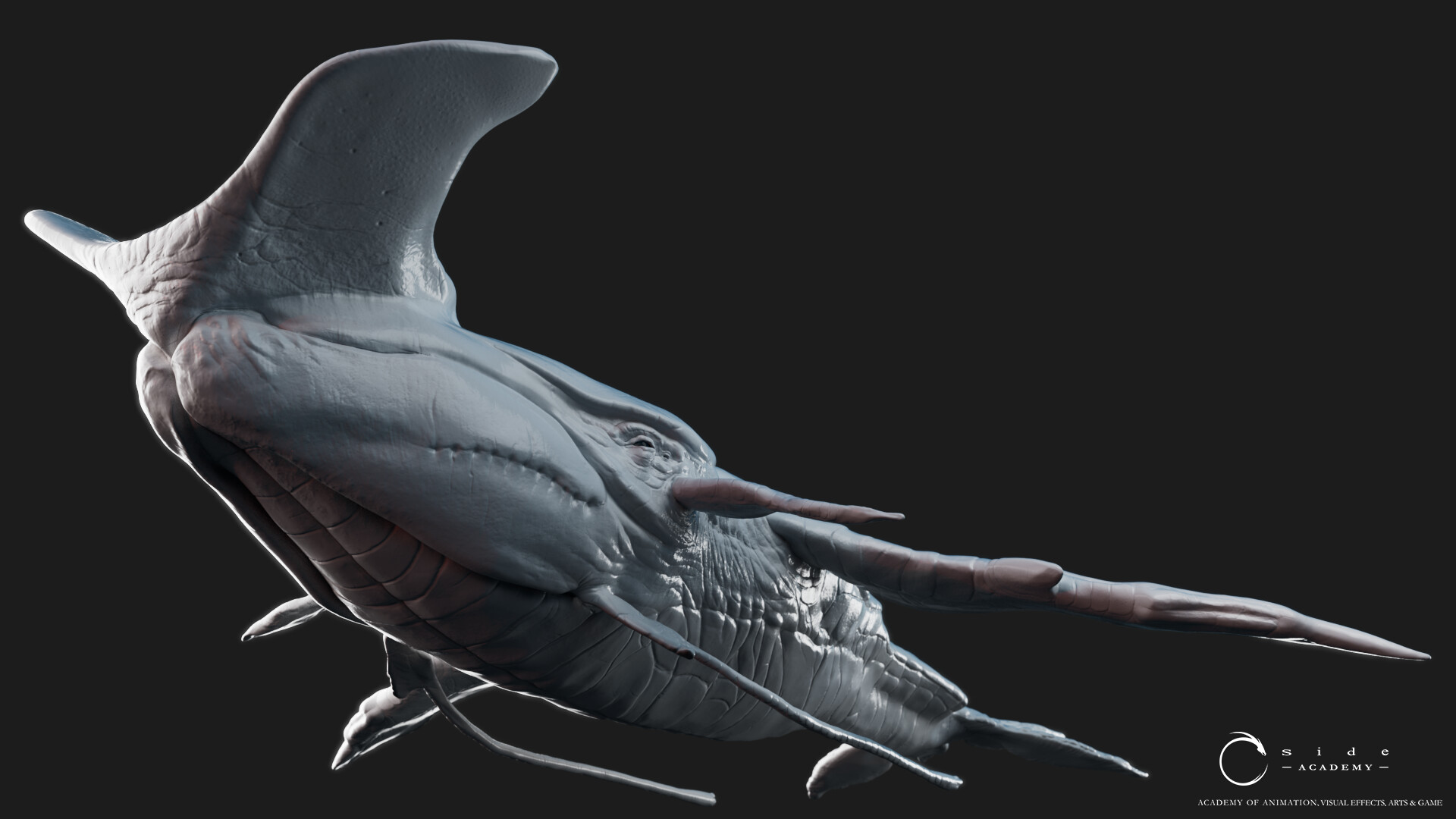The image features a computer-generated, light gray creature resembling a hammerhead shark against a solid black background. The perspective is from beneath, showcasing the underside of its head and body, with detailed texture giving it a 3D appearance. The creature has distinctive anvil-like horns and sharp fins protruding from its sides. The left side of its body and eye are visible, accentuated by focused lighting and shading on the upper left. At the bottom right of the image, text reads “Side Academy of Animation, Visual Effects, Arts, and Games,” accompanied by a circular logo with a swoosh.